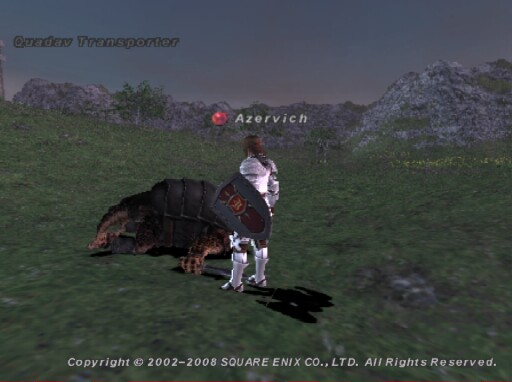In this screenshot from a video game, the central focus is a character clad in intricate armor, holding a dark burgundy and black shield emblazoned with an emblem, facing the viewer. The character gazes downward upon an armored creature with a dark brown body, resembling an animal. The scene is set in a lush grass field with majestic gray mountains in the background, under a moody, bluish-gray sky. At the bottom of the image, a text overlay reads, "Copyright 2002-2008, Square Enix. All rights reserved."